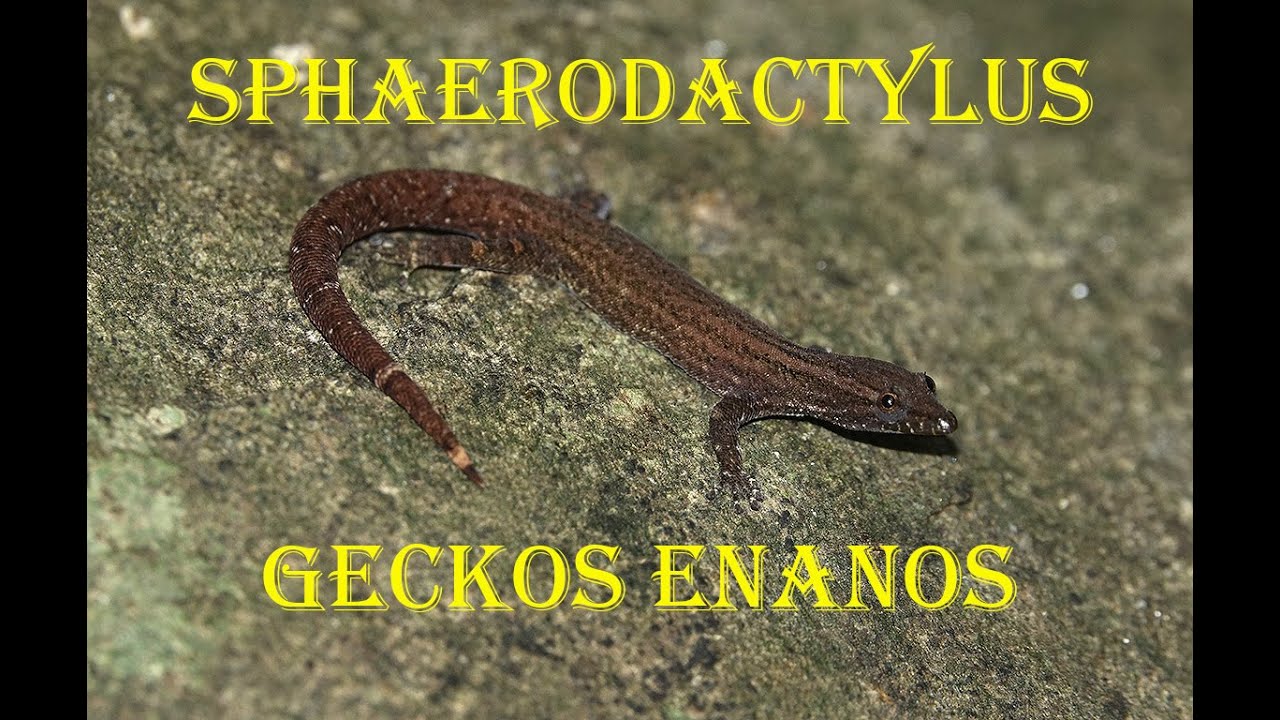The image captures a detailed view of a small brown lizard, a specific type of gecko, lying on a grayish, rocky surface with a subtle green texture. The environment appears rugged yet smooth. The gecko's slender body is adorned with darker brown horizontal stripes and culminates in a long, pointy tail with intermittent white stripes and a hint of yellow towards the end. The creature, facing to the right, has a triangular-shaped head, small, black eyes, tiny front legs, and short back feet. Above the gecko, in bold yellow capital letters, the word "S-P-H-A-E-R-O-D-A-C-T-Y-L-U-S" is prominently displayed, while below it, the words "G-E-C-K-O-S" and "E-N-A-N-O-S" are similarly printed, indicating the specific species.